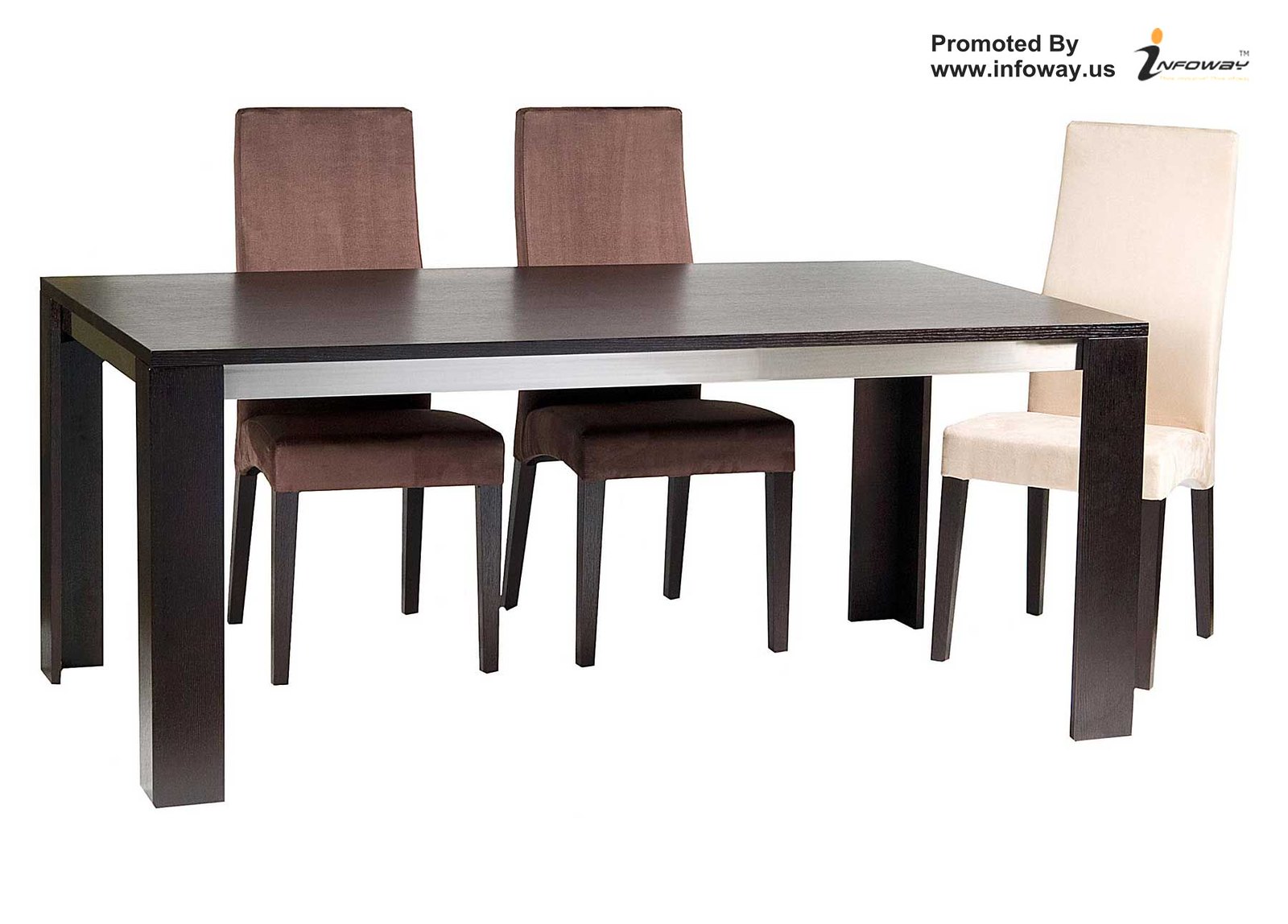This image appears to be a computer-generated ad for office or dining room furniture, featuring a long oblong table and three chairs. The table has a dark, almost black, brown color with thick rectangular legs and a metal trim. It is designed to comfortably fit six to eight people but currently has only three chairs placed around it. Two of these chairs are brown with black legs, and the third is white with black legs, forming a consistent design style. The chairs are tall-backed and covered in a felt-like material. The white chair is positioned at the head or foot of the table at an angle, while the two brown chairs are placed along the long side, facing the photographer. The image includes a note in the top right corner indicating it is "Promoted by www.infoway.us," suggesting that Infoway.us is the promoting entity, possibly an office supply company.